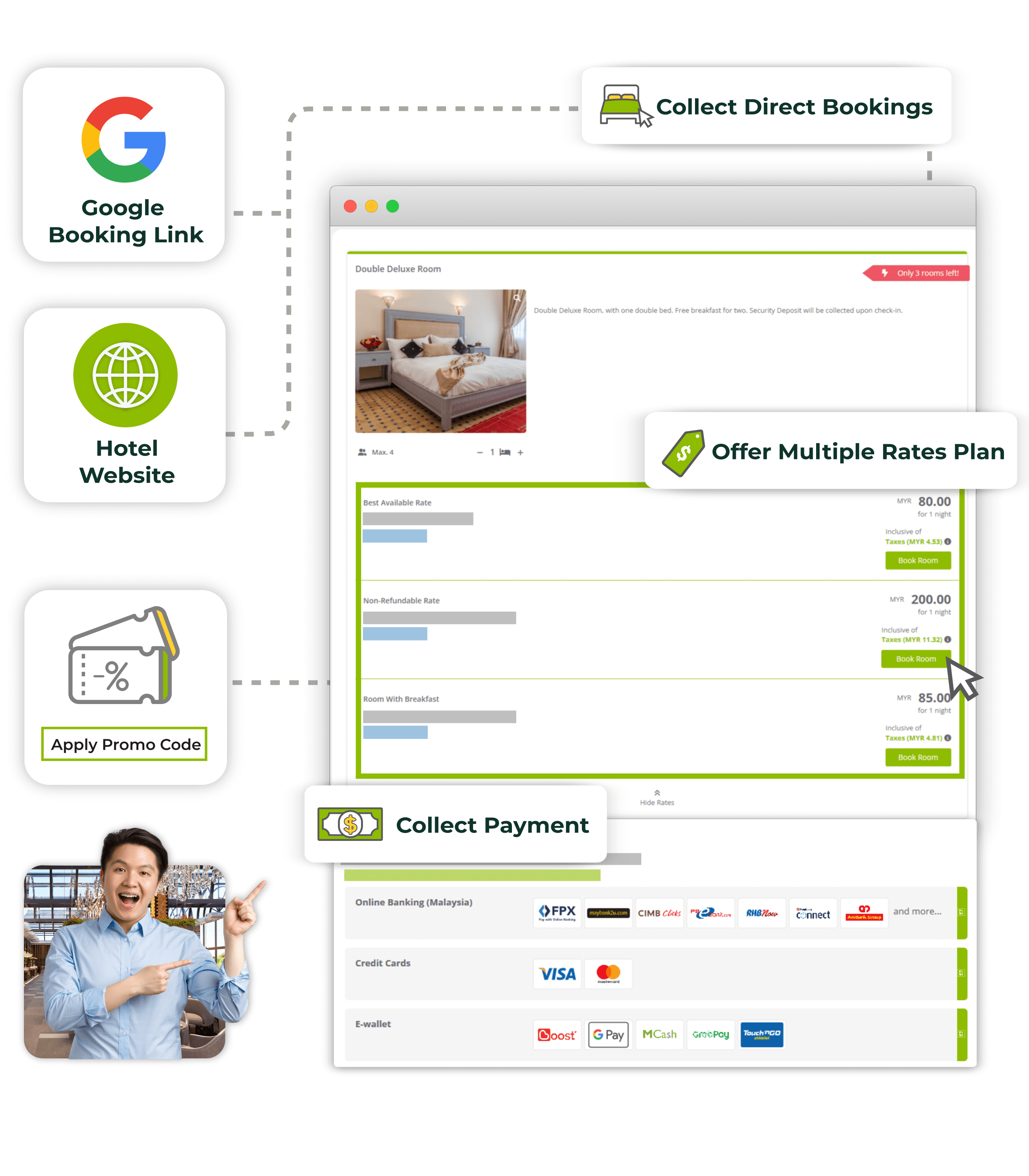In this image, an advertisement for booking a hotel is prominently displayed. On the left side, the text "Google Booking Link" is clearly visible alongside the recognizable Google logo, indicating a direct booking service. Beneath this, there are two separate boxes labeled "Hotel Website" and "Apply Promo Code," suggesting options for navigating to the hotel's official site or inputting discount codes.

At the bottom of this section, a man with short dark hair, dressed in a blue shirt, is depicted pointing upwards towards the boxes, presumably drawing attention to the booking options. To the right, the heading "Collect Direct Bookings" is easily noticeable at the top, emphasizing the purpose of the advertisement.

Below this heading, an image of a hotel room labeled "Double Deluxe Room" is presented, suggesting the type of accommodation available. The cost options are listed beneath the room image: "Best Available Rate $80," "Non-Refundable Rate $200," and "Room with Breakfast $85." However, some of the information near these rates appears to be blurred or obscured.

At the bottom of the right section, a segment titled "Collect Payment" is visible, showcasing various payment options for finalizing the booking. This detailed depiction aligns with the overall theme of promoting direct hotel bookings through an intuitive and engaging interface.